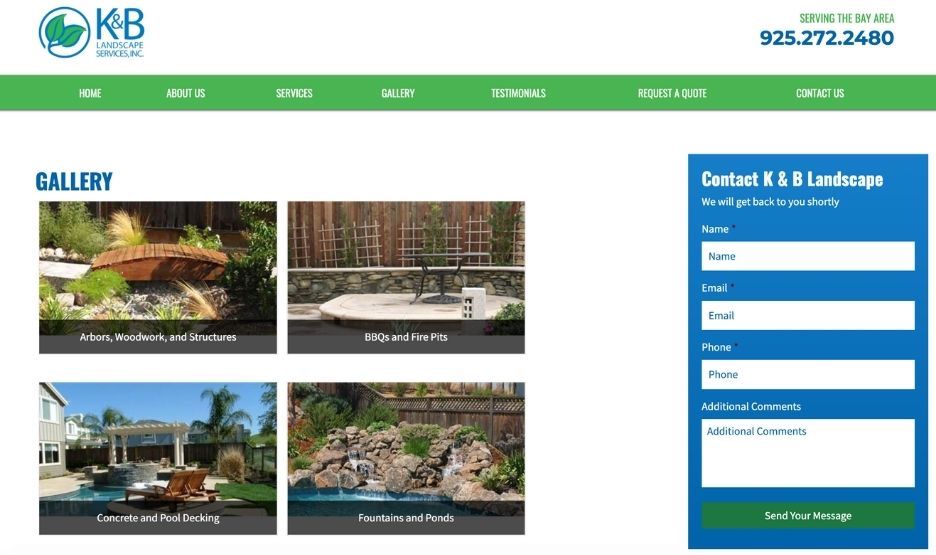The website for K&B Landscape Services Inc. prominently features a well-organized layout. In the upper left corner, the logo showcases the initials "K&B" with a small ampersand nested between the "K" and "B." Adjacent to the logo, two green leaves are encapsulated within a blue circle. Positioned to the right of the website, the phrase "Serving the Bay Area" is displayed alongside the contact number, 925.272.2480. 

A medium-shaded green bar with a slight drop shadow extends across the top of the page, housing the main menu with options: Home, About Us, Services, Gallery, Testimonial, Request a Quote, and Contact Us, all in white text. Below this navigation bar, a blue header clearly labels the section as the "Gallery."

The gallery section features four outdoor images:
1. The first image depicts a picturesque bridge.
2. To the right, there's a raised platform furnished with a table and a small stone wall behind it.
3. Below that, another image features a gazebo, possibly accompanied by a hot tub or an elevated area surrounding a pool.
4. Finally, the last image on the right showcases a captivating rock feature with a small waterfall cascading into a pool.

Each photo contains descriptive text on translucent overlays:
- Top left: "Arborist, Woodwork and Structures"
- Top right: "Barbecues and Fire Pits"
- Lower left: "Concrete and Pool Decking"
- Lower right: "Fountains and Ponds"

On the right side of the page, within a blue field, there's a contact section labeled "Contact K&B Landscape, we'll get back to you shortly." This area includes fields for Name, Email, Phone, and Additional Comments, each duplicated in white input fields. The blue background extends lower than the photos on the left, and at the bottom, a green button labeled "Send Your Message" is available for submissions.